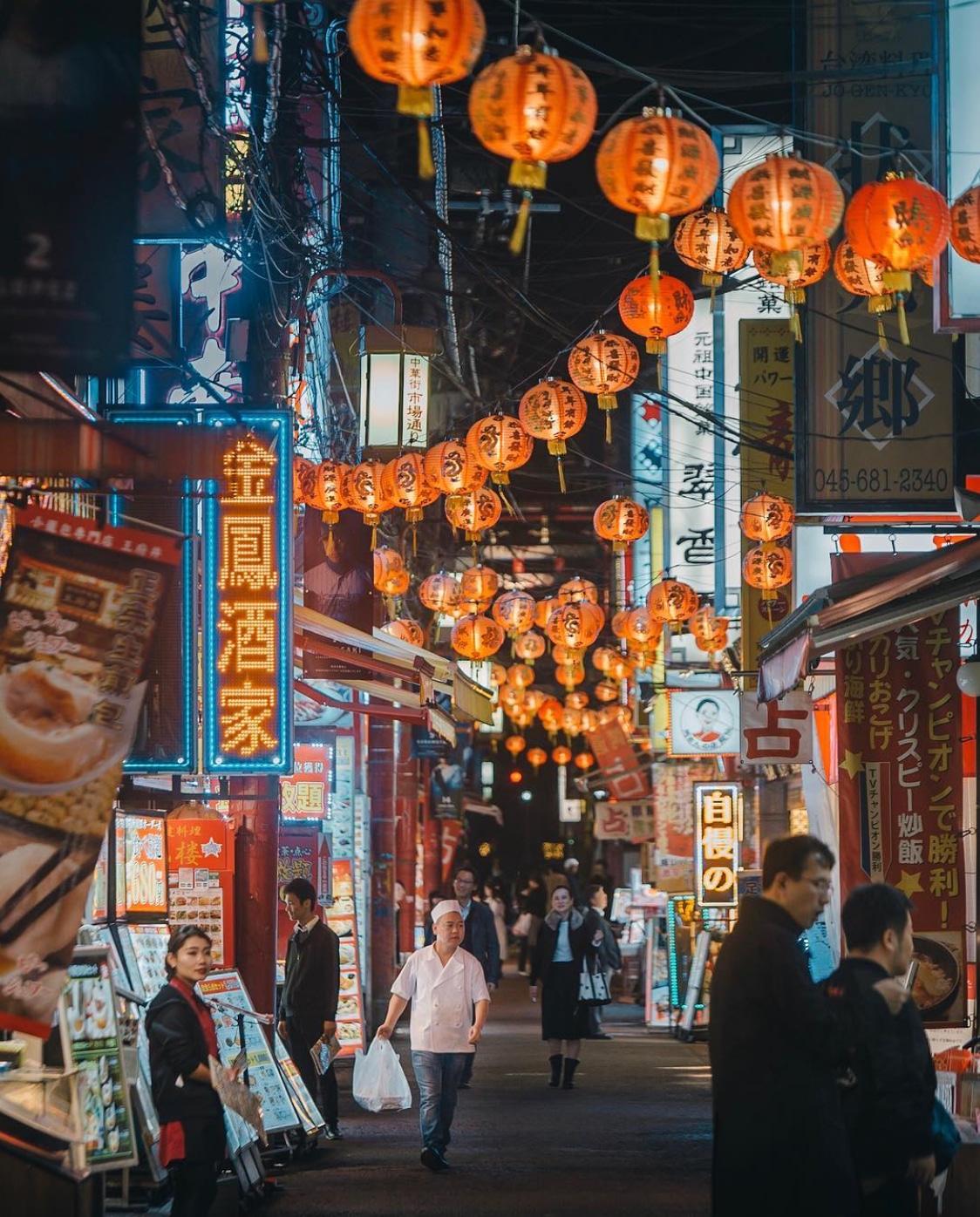This vibrant color photograph captures a bustling nighttime street scene in an Asian city, possibly in Japan or China. The narrow pedestrian street is lined with a variety of shops and restaurants adorned with bright neon signs and vertical banners displaying Chinese characters. The atmosphere is festive, with several rows of orange, globe-shaped paper lanterns strung in a zigzag pattern overhead, casting a warm glow across the street filled with oranges, reds, and blues.

The street itself is dark pavement, crowded with pedestrians. Most are walking toward the camera, perusing the food stalls and market booths that flank the walkway. Central to the image is a man dressed in a white chef's hat, a matching white shirt, and blue jeans, holding a plastic bag that appears to contain food containers. His attire suggests he might be a cook or vendor. Behind him, a woman looks towards the camera, while two men in dark suits stand to the bottom right, peering into a stall.

The lively ambiance, coupled with the neon-lit signs and paper lanterns, paints a vivid picture of a traditional yet modern Asian night market teeming with life and activities.